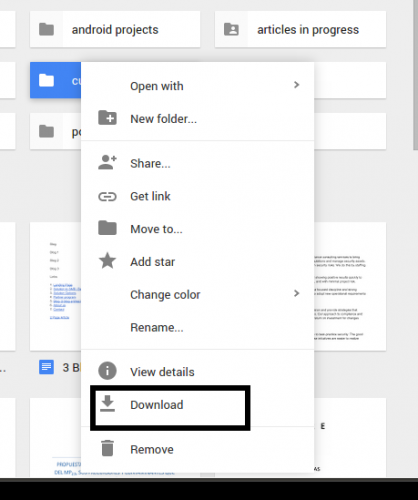Screenshot Description: An Android phone screenshot displaying a user interface for managing files. At the center of the screen, there is a pop-up menu overlay, titled "Open With," allowing the user to select an application for file opening. This menu contains various options, including "New Folder," "Share," "Get Link," and "Move To." Additional choices such as "Add a Star" and "Change Color" (with a drop-down list for color selection) are visible, as well as "Rename," "View Details," "Download," and "Remove." The "Download" option is prominently highlighted with a thick border, indicating the user's active selection. 

Behind the pop-up menu, the main file management screen is partially visible. The screen is divided into two main sections: "Android Projects" on the left, and "Articles in Progress" on the right. At the top, there is a header with alternating colors. Below this header, a list of files is displayed, with one file actively selected, triggering the aforementioned pop-up menu. Additional files are listed underneath the selected file, though their details are obscured by the overlay. The user appears to be in the process of choosing whether to download the selected file or perform another action.

Overall, the image illustrates the functionality and design of an Android file management system, highlighting the user’s interaction with file options via a context menu.